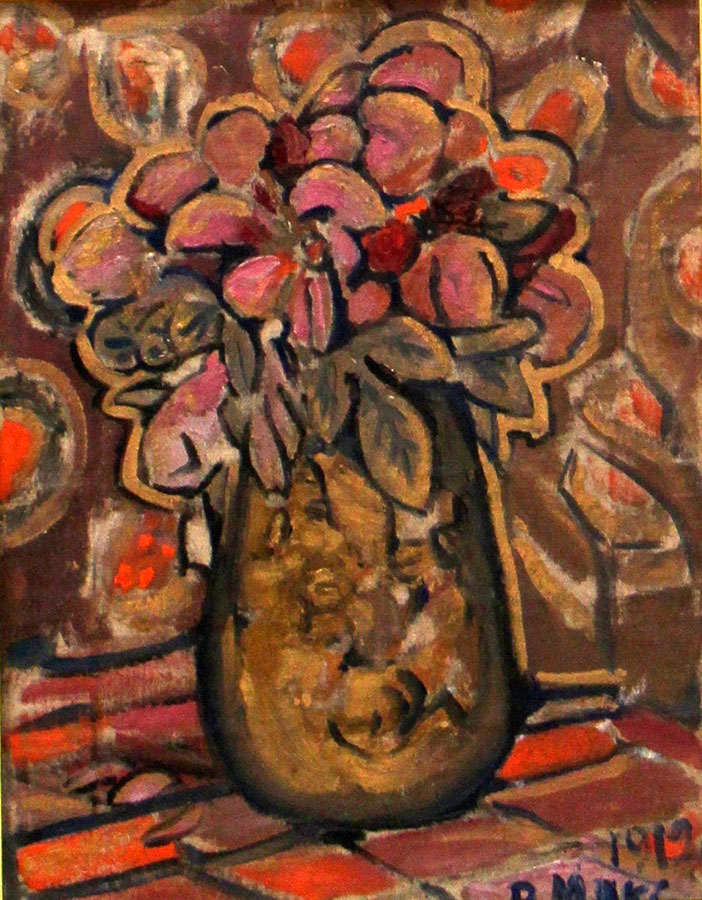The painting depicts a vase of flowers resting on a tiled surface. The vase itself is a tannish brown color with a curved shape that becomes narrower towards the top. The flowers in the vase are predominantly pink and red with some burgundy hues, but lack intricate details in the petals, giving them a more rounded and simplistic appearance. Some green leaves are visible, including a distinct set of three that drape over the edge of the vase. The tiles beneath the vase feature a checkered pattern of red and burgundy shades.

In the background, there is a murky brown wallpaper adorned with various circles and dots of red, adding depth and texture to the scene. The overall color palette of the painting is dominated by reds, browns, and greens, creating a warm and earthy tone. A signature is visible at the bottom, along with the date "1919" in the lower right corner.